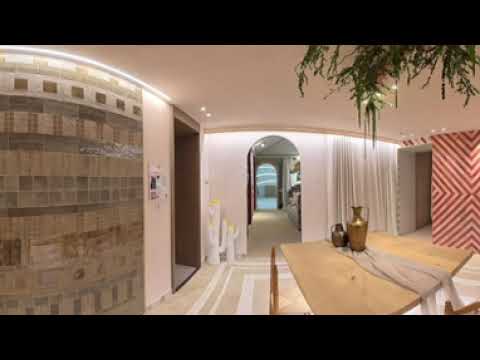The image depicts the interior of a beach house with a unique blend of styles. Dominating the right side is a wall adorned with a red and white geometric design. A light wood table sits in the foreground on the right, draped with a beige cloth. Atop the table, a dull gold pitcher and a smaller silver bottle catch the eye. The beige and white floor complements the monochromatic beige walls, which feature textured or mosaic patterns reminiscent of Middle Eastern or Egyptian art. 

Suspended in the upper right corner, green leafy branches introduce a natural element, seemingly intruding into the indoor space. Toward the left, another wall exhibits a brownish tile mosaic pattern, evoking an ancient pyramid aesthetic.

The central portion of the image leads the eye down a hallway toward an ambiguous light source, possibly another room or the outdoors. Adjacent to this hallway, on the right, hangs a white curtain beside what might be a bathroom door. The scene is framed by medium-thick black borders at the top and bottom, and overall, the room feels spacious albeit slightly blurred, as if viewed through a pixelated filter.